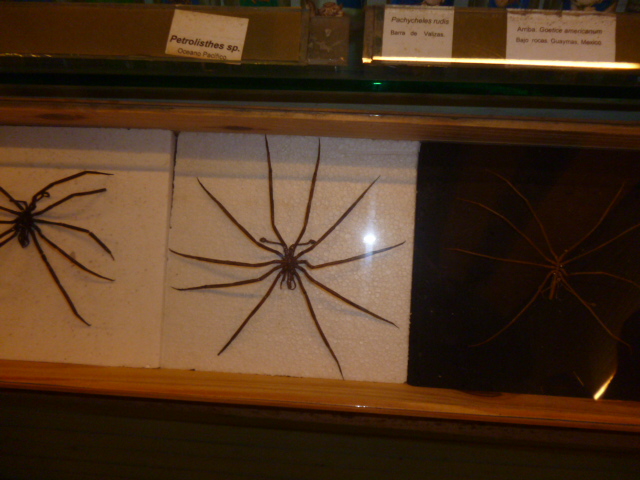The image depicts a detailed display of three large spiders in a collector's case. Positioned within a brown wooden frame, the display is organized into three sections. The two spiders on the left are mounted on white slabs, with a light brown laminate board beneath them. The spider on the right, barely visible against its dark background, is also included in the collection. These arachnids are characterized by their long legs and small bodies, with the middle spider resembling a starfish and the left one appearing slightly crumpled. Above the display case, there are out-of-focus white cards, likely containing typed information about the spiders, such as their names. The overall color palette of the image includes shades of brown, white, and black. The display seems to be horizontal, rather than mounted on a wall, suggesting a close-up view of a carefully curated collection.